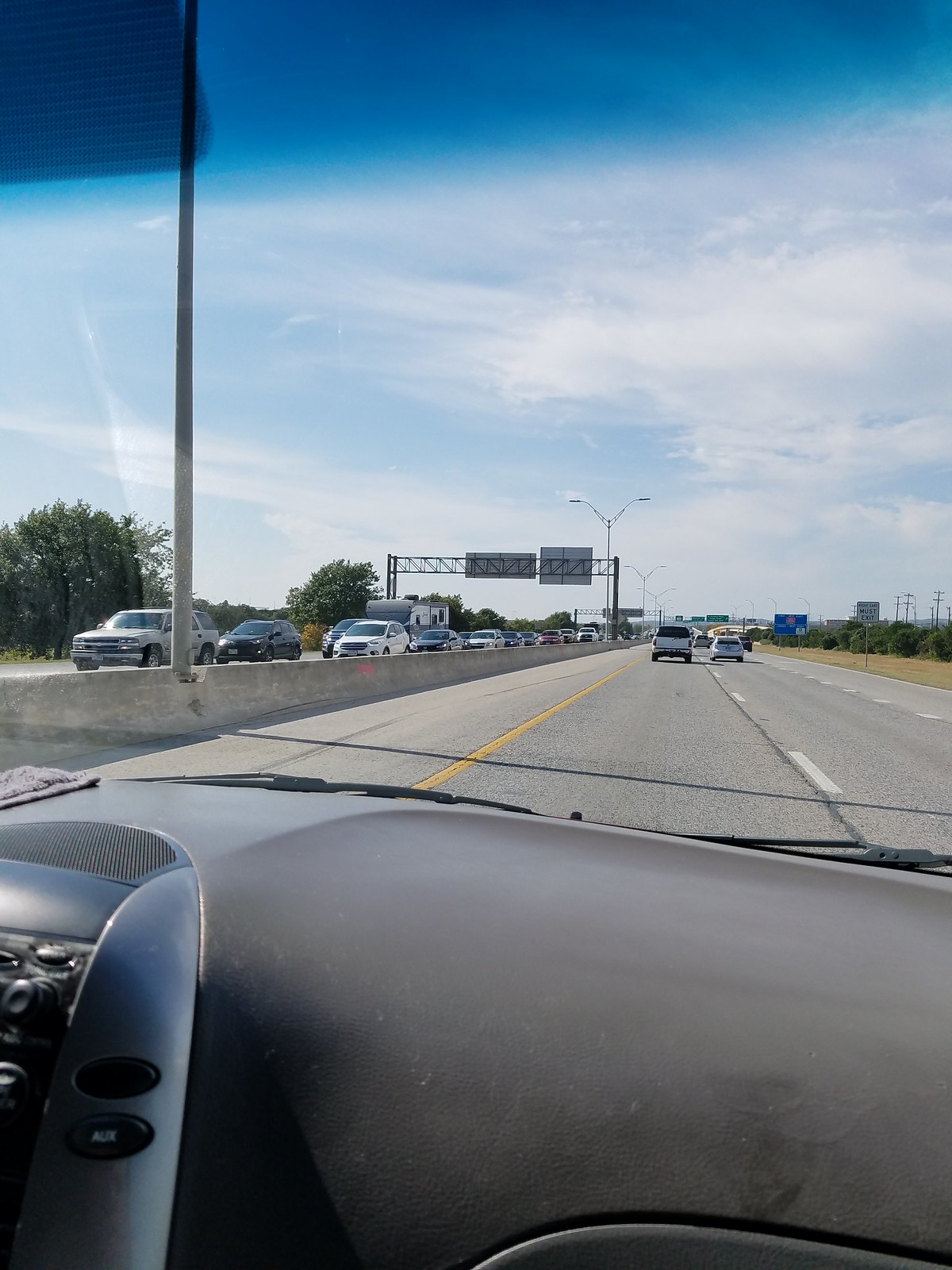This photograph, taken from the passenger seat of an older car, provides a detailed view of a three-lane freeway. The foreground reveals the gray dashboard, featuring silver buttons likely for heat and temperature controls, and a portion of the center console. The vehicle is traveling in the far left lane, adjacent to a concrete median, marked by a solid yellow line. To the right is the center console with typical dashboard features, and to the left, the windshield wipers are visible.

The freeway, appearing with faded gray pavement, has oncoming traffic in the opposite direction, separated by a concrete barrier with trees and vegetation on either side. There is heavy traffic on the opposite side, including various cars and a camper. Towards the left, there is a prominent lamppost on the median, and in the distance, a large metal pole and the backs of exit signs mounted on a metal truss are visible. The scene is framed by trees and vegetation flanking both sides of the road.